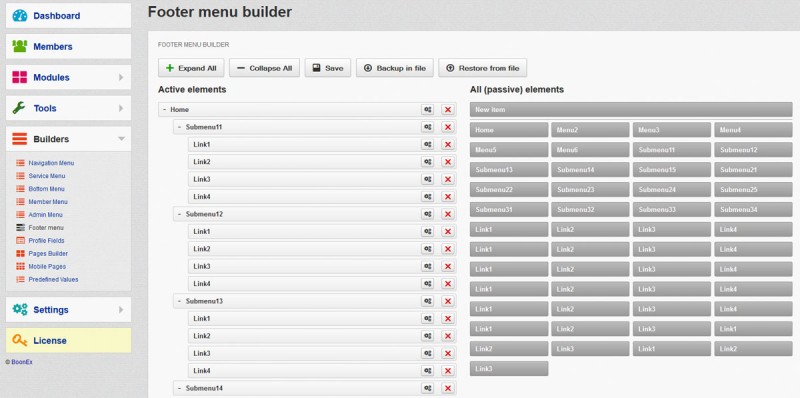The image is a screen capture of an app interface, showcasing its layout and various features. The app screen is divided into two main sections: a vertical navigation pane on the left and a larger content area to the right.

At the top of the screen, a header with a gray background displays the text "Footer Menu Builder" in black. Below this header, the left vertical pane is organized into several menu items, each displayed on a white rectangular background. Starting from the top, these items are labeled: "Dashboard," "Members," "Modules," "Tools," and "Builders." 

Underneath the "Builders" section, there are multiple options written in blue text, although their specific titles are not indicated in the provided description. Additionally, towards the bottom of the vertical pane, there are two more menu options titled "Settings" and "License," which are highlighted with blue text on a yellow background.

The larger right section features various horizontal bars in off-white and gray colors, although their specific content or functionality is not detailed. This right section appears to be the workspace where the main app activities take place, possibly related to the builder tool indicated in the header.